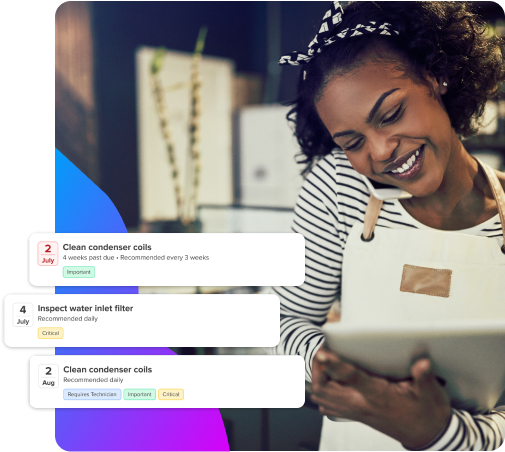This is a detailed screenshot of what appears to be a calendar app. The background features a photograph of an African American woman who seems to be a clerk or a staff member. She is engaged in a phone conversation, with her head tilted to the left, while holding a tablet. The woman is dressed in a long-sleeve striped shirt and a white apron with a black patch in the middle, suggesting she is in a professional environment, potentially a restaurant or retail store. She appears to be multitasking, possibly discussing something with a customer while inputting data into her tablet.

Overlaying the image are three semi-transparent boxes positioned on the left side of the screen, each containing task reminders and their respective tags:

1. **Box 1 (July 2)**: A reminder to clean the condenser coils, which is noted to be four weeks past due and recommended to be done every three weeks. This task is marked with an "Important" tag in green.
   
2. **Box 2 (July 4)**: A reminder to inspect the water inlet, recommended to be checked daily. This task holds a "Critical" tag in yellow.
   
3. **Box 3 (August 2)**: Another reminder to clean the condenser coils, this time recommended daily. This task carries three different tags: "Requires Technician" in blue, "Important" in green, and "Critical" in yellow.

These tags highlight the urgency and importance of the tasks, helping the user prioritize their responsibilities.